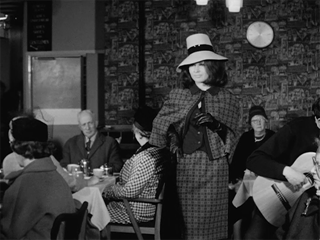In this black and white photograph, we see a scene that appears to be from the 1930s or 40s, potentially in a restaurant or a hotel setting. Dominating the center of the image is a young woman with shoulder-length dark hair, wearing a long plaid skirt and a white sun hat adorned with a black stripe. She is staring directly at the camera, capturing our attention. Surrounding her, people are seated at tables to the left and right, dressed in period-specific clothing—men in suits and women in dresses and hats. There's an older man, possibly in his 80s, slumped over a table, indicating a moment of either rest or deep thought. Another woman in fancier, perhaps more modern attire for the era, wearing a hat and black gloves, is seen walking through the scene. Adding to the ambiance, a man dressed in a black shirt is playing an acoustic guitar, filling the air with music. The overall atmosphere suggests a fancy dinner or an event, set against a backdrop of a brick wall with various hues of grey, contributing to the nostalgic, almost cinematic quality of the image.